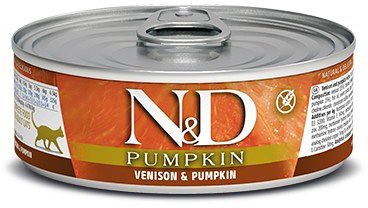This photograph showcases a can of N&D cat food, distinctly set against a pristine white surface and backdrop which accentuates its details. The small, cylindrical can is equipped with a silver pull-top lid, ensuring easy access to its contents. The label itself is a vibrant blend of colors and clear typography. The brand name 'N&D' is prominently displayed in white against a bold orange segment. Beneath it, the flavor 'Pumpkin' is elegantly written in white on a golden stripe, while 'Venison & Pumpkin' appears just below on a contrasting white background.

A significant feature of the label is a white section adjacent to the primary branding area, adorned with a refined gold silhouette of a cat, adding a touch of elegance and visual interest. On the opposite side of the can, detailed nutritional information is provided, listing ingredients and other essential dietary insights, underlining the product’s comprehensive approach to pet nutrition. This meticulous arrangement augments the can's overall appeal, presenting it not just as a mere product but as a carefully crafted item designed for discerning pet owners.